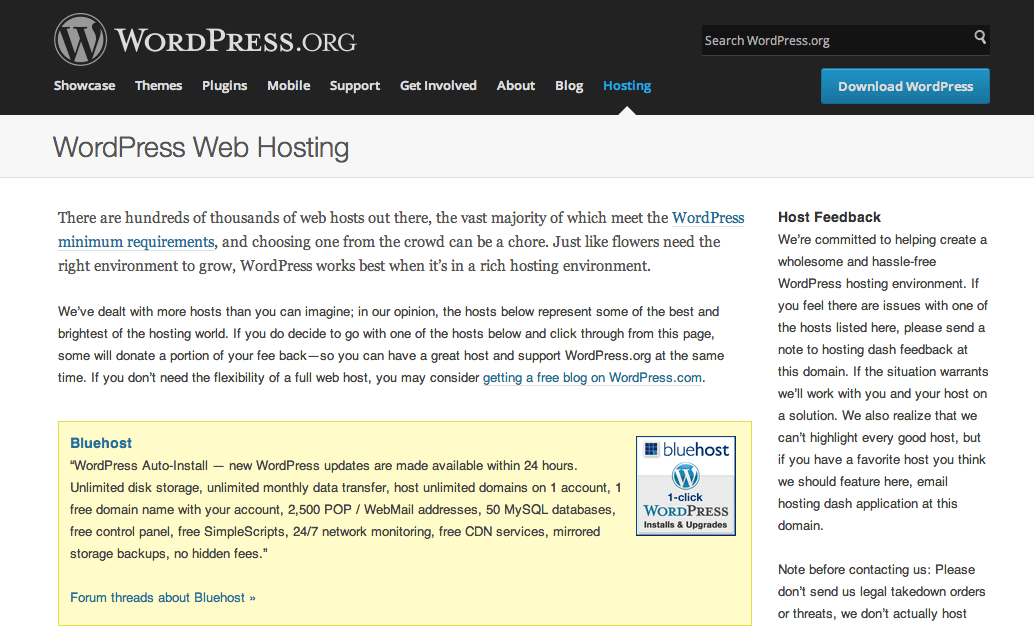The image shows the WordPress.org homepage, specifically focused on the Hosting tab. In the top left corner, the WordPress.org logo, featuring the iconic "W," is prominently displayed. The navigation bar stretches across the top, listing several options: Showcase, Themes, Plugins, Mobile, Support, Get Involved, About, Blog, and Hosting, with the latter being selected.

Underneath the Hosting tab, the page details "WordPress Web Hosting," emphasizing the abundance of web hosts that meet the minimum WordPress requirements and the importance of a rich hosting environment for optimal performance. A prominent advertisement for Bluehost is displayed, indicating a partnership between WordPress and Bluehost. This is highlighted by a banner in the lower right corner, where the Bluehost logo is accompanied by WordPress branding and the phrase "OneClick," suggesting a seamless integration for users. The text explains that users can purchase their own website through Bluehost, obtaining a custom URL instead of a standard WordPress.org address.